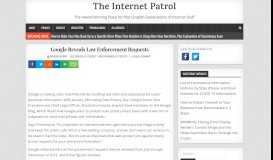The image depicts a detailed screenshot of a webpage from an article titled "The Internet Patrol." Directly beneath the title, there is a line of text that remains illegible. Below this text is a horizontal gray bar with numerous buttons on the left side, serving as navigation tabs for the website. Beneath this navigation bar, the article begins with a prominent header followed by several descriptive bullet points before delving into the main paragraphs of text.

Additionally, pixelated social media symbols are visible, with the most recognizable ones being the icons for Facebook and the old Twitter logo. On the right side of the page, a white rectangular section contains three paragraphs of text. Flanking this section are vertical gray bars. Along the far right edge of the image, there is a thin, solid black line extending from the top to the bottom of the page.